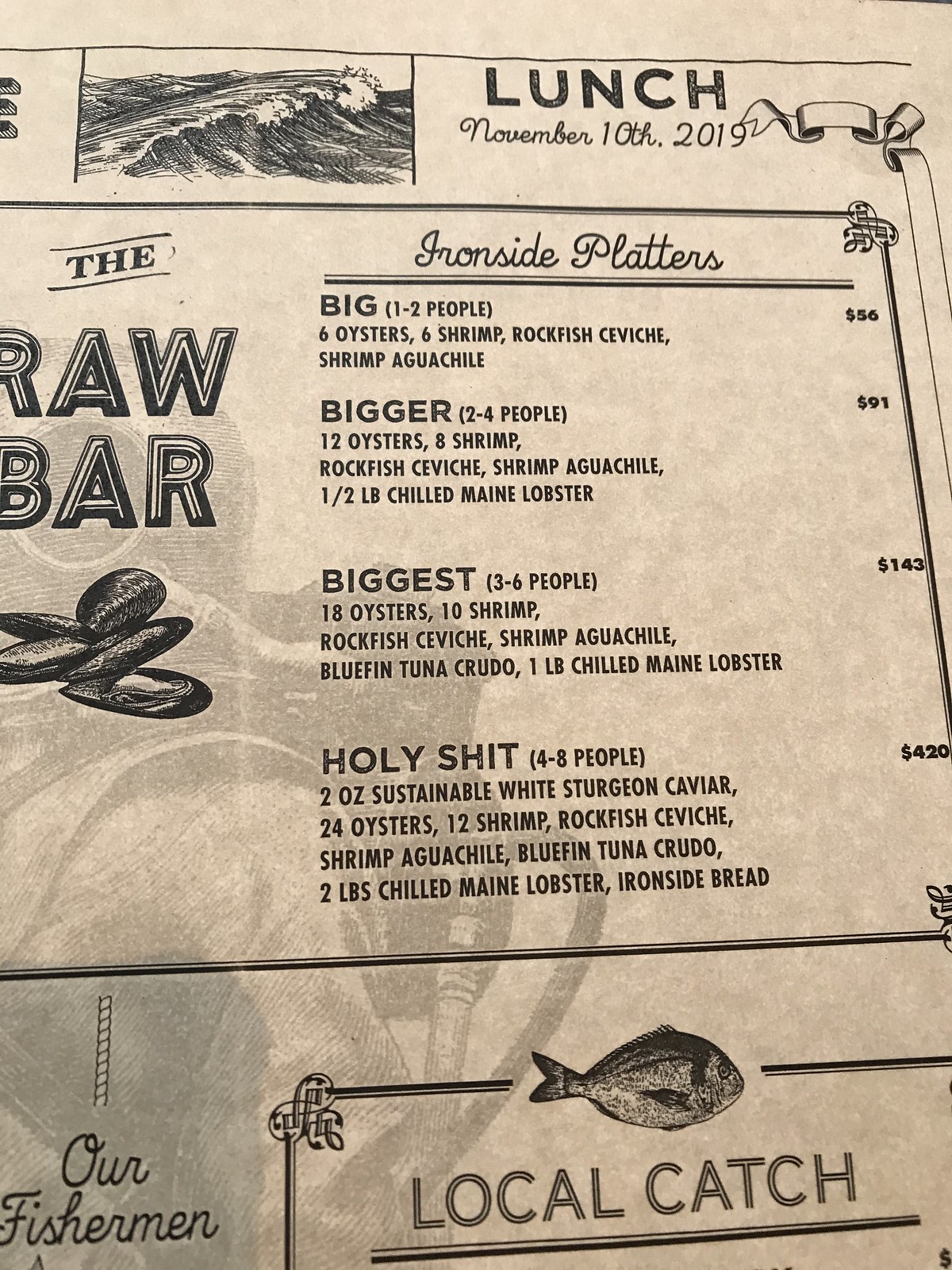Here's a detailed and cleaned-up caption for the image:

---

This image features a seafood restaurant menu with a light brown, almost beige background, and black text and designs. In the upper left corner, there is a decorative line with hand-drawn waves beneath it, accented with white highlights to simulate choppy waves. To the right of this, in bold black letters, is the word "Lunch," underneath which the date "November 10th, 2019" appears in smaller font. A small ribbon emblem runs vertically along the right edge of the menu but is partially cut off.

On the far left side, the section titled "The Raw Bar" is prominently displayed in large, black, 3D-outlined letters. Below this heading, black illustrations of clam or oyster shells with visible white interiors are depicted.

On the right side of the menu, various "Ironside Platters" are described with the following details:

- For one to two people: Six oysters, six shrimp, rockfish ceviche, shrimp aguachile. Price: $56.
- For two to four people: Twelve oysters, eight shrimp, rockfish ceviche, shrimp aguachile, half a pound of chilled Maine lobster. Price: $91.
- For three to six people: Eighteen oysters, ten shrimp, rockfish ceviche, shrimp aguachile, bluefin tuna crudo, one pound of chilled Maine lobster. Price: $143.
- For four to eight people ("Holy Shit"): Two ounces of sustainable white sturgeon caviar, twenty-four oysters, twelve shrimp, rockfish ceviche, shrimp aguachile, bluefin tuna crudo, two pounds of chilled Maine lobster, IronSide bread. Price: $420.

There is a horizontal line toward the bottom, below which the section titled "Local Catch" appears, accompanied by the phrase "Our Fishermen" on the left. There's an indistinct drawing in the background.